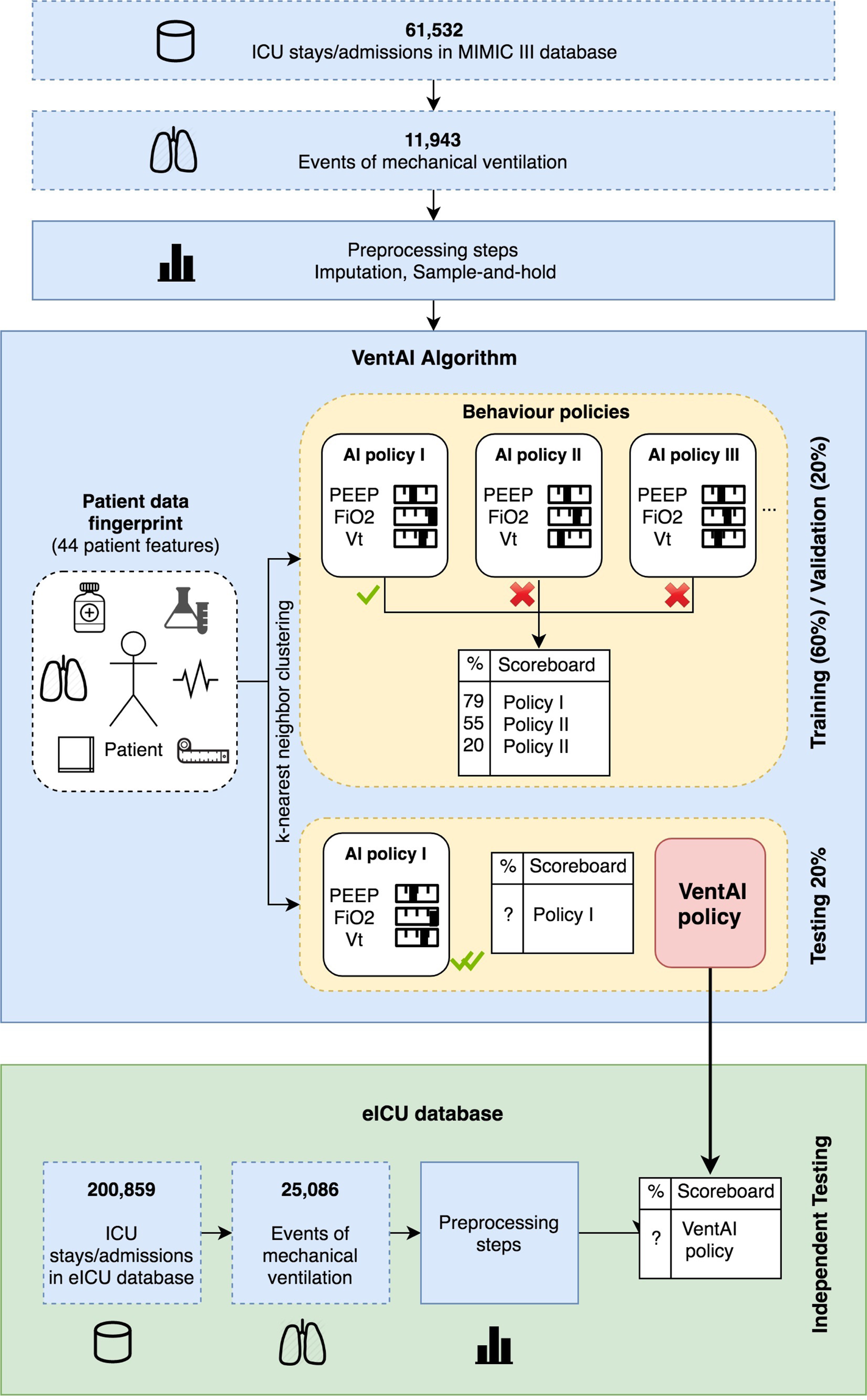The image depicts a detailed flowchart of an event AI algorithm focused on ICU patient data. At the top, there are 61,532 ICU stays/admissions recorded in the MIMIC-III database. An arrow points to the next section indicating 11,943 events of mechanical ventilation. The flow follows preprocessing steps such as imputation and sample-and-hold techniques. Central to the diagram is the event AI algorithm, which is illustrated within a large square featuring behavior policies (AI Policy 1, 2, and 3) on a pale salmon pink background. Evaluation results are provided below, showing AI Policy 1 scoring 79%, Policy 2 at 55%, and Policy 3 at 20%, with corresponding check marks and X marks indicating their efficacy.

To the left, the diagram details a black-text labeled "patient data fingerprint," which includes a stick figure surrounded by images representing 44 patient features, such as medication, lungs, pulse, heart rate, scientific bottles, and a tube. At the bottom, the eICU database section is defined with three blue squares summarizing 200,859 ICU stays/admissions and 25,086 events of mechanical ventilation, coupled with preprocessing steps. The overall visual, combining blue, green, and pale peach highlights, outlines the integration of patient data and AI-driven behavioral policies for improving ICU care.